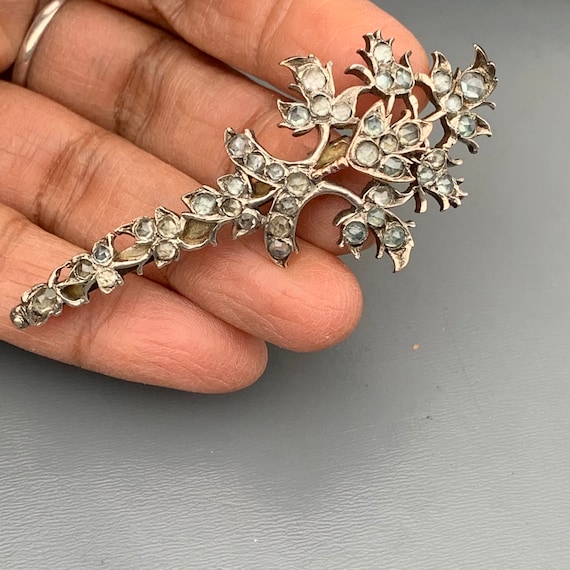In this indoor photograph, a left hand with light brown skin and a silver ring on the middle finger is seen emerging from the upper left corner, against a gray vinyl background with subtle wavy lines. The fingers are delicately holding a long, silver decorative brooch resembling a sword. This Victorian-style brooch, likely antique, is embellished with numerous small, diamond-like gems arranged throughout. The top right portion of the brooch flares out into a decorative vine and flower pattern, while the bottom narrows into a more streamlined, sword-like shape. The brooch appears to have a clip on the back, suggesting it can be fastened to clothing or other fabric.